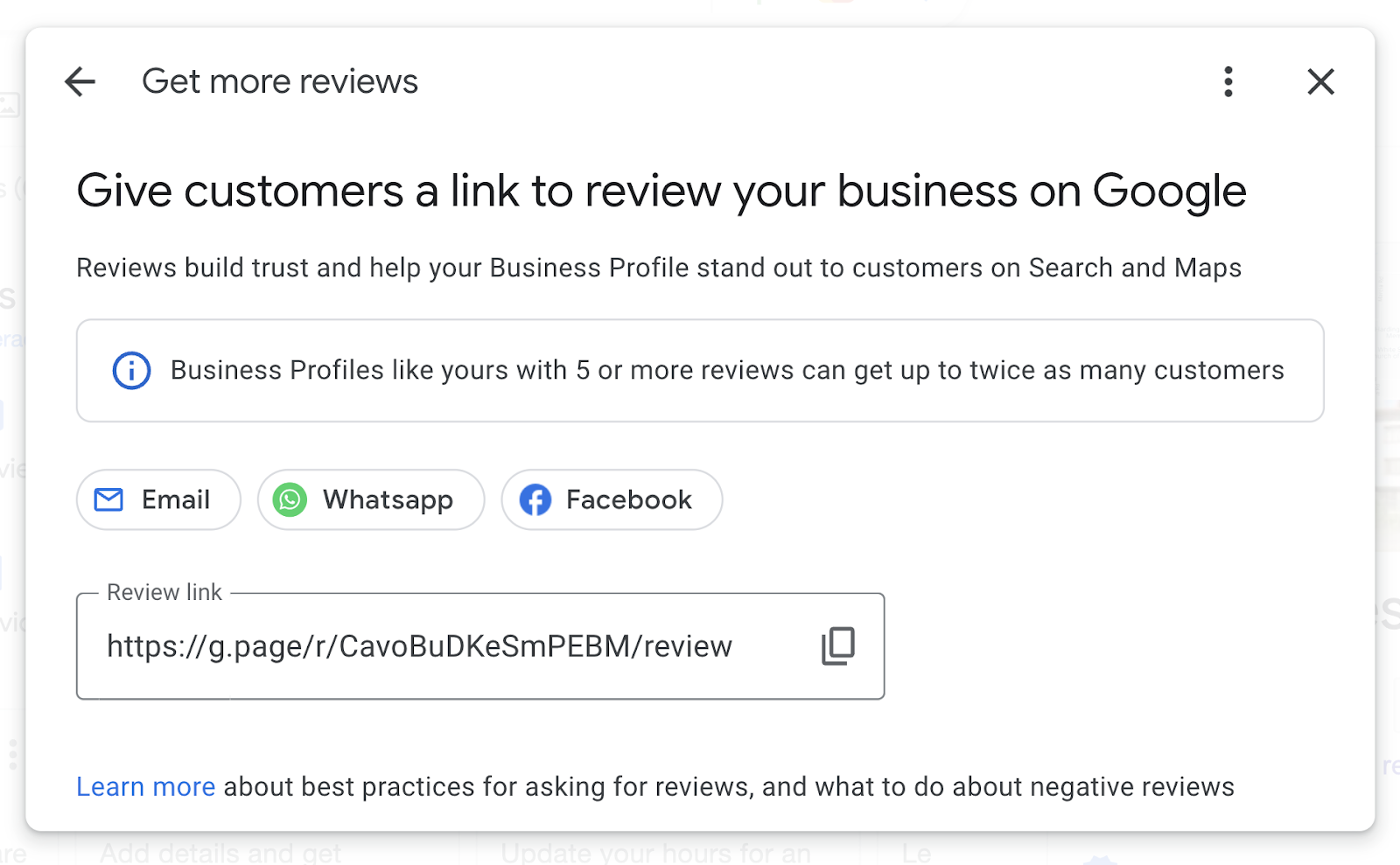In this image, a text box is prominently displayed with the primary message "Get More Reviews", accompanied by an arrow pointing to the left. Below this, additional text reads: "Give Customers a Link to Review Your Business on Google. Reviews build trust and help your business profile stand out to customers on Search and Maps."

Further down, the text emphasizes that "business profiles like yours with five or more reviews can get up to twice as many customers." Below this, there are text bubbles labeled for different platforms: Email, WhatsApp, and Facebook.

Next, a highlighted section labeled "Review Link" features a URL: https://g.page/r/cavoBUDKESMPEVM/review with a symbol adjacent to it indicating the option to copy the link.

At the bottom, in blue text, the link "Learn More" is visible, followed by the black text "About Best Practices for Asking for Reviews and What to Do About Negative Reviews."

The entire content is displayed within a white text box, with the majority of the text appearing in black for clarity and emphasis.